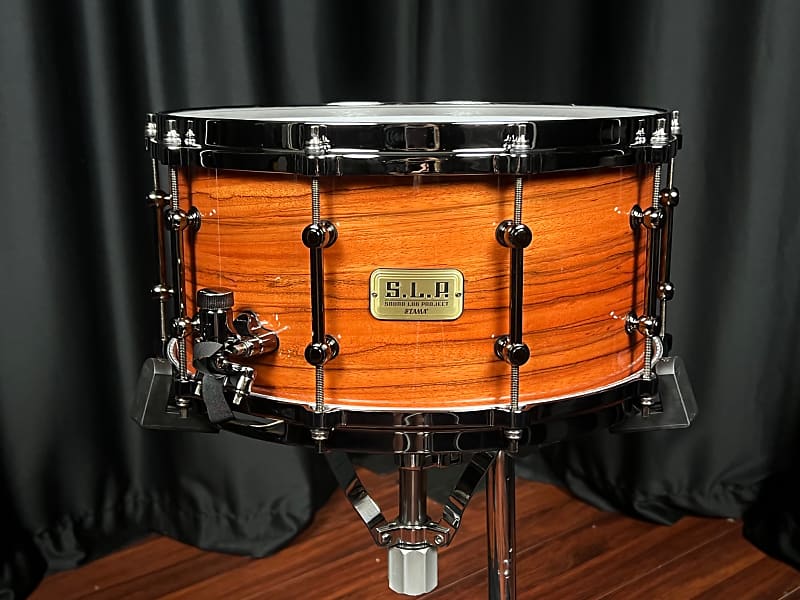This detailed color photograph features a beautifully crafted drum, prominently displayed on a dark wooden surface. The drum is supported by a sturdy metal framework, enhancing its elegance and stability. The drum's body is constructed from polished wood, exuding a rich, warm tone that complements its sophisticated design. Encircling the upper rim, polished metal accentuates the drum's structure, with numerous vertical metal supports further reinforcing its build.

A gold tag situated at the center of the drum proudly displays the brand "SLP," followed by partially legible text and the word "PROJECT." Below this, the inscription "S-T-A-M-A" can be seen. The backdrop features shiny black curtains that cascade down to the floor, adding a touch of dramatic contrast to the scene. The photograph is devoid of people, animals, and plants, allowing the viewer's focus to remain entirely on the striking drum.